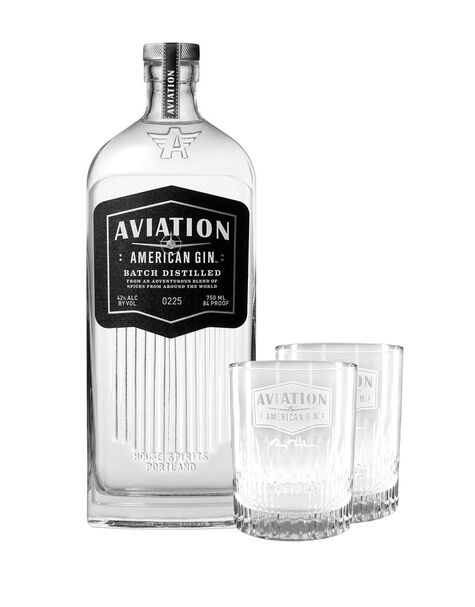The image showcases a meticulously clean, square-shaped, clear glass bottle of Aviation American Gin, prominently placed against a plain white background. The bottle stands approximately three to four inches high and features a straight neck that flares gently towards its base. The neck is capped with a metallic silver, tamper-proof seal adorned with a black and white label that reads "Aviation," and bears a distinctive emblem of an "A" with outstretched wings. 

The front of the bottle is distinguished by a black label with white lettering that reads: "Aviation American Gin, batch distilled." Below this, additional details are included, specifying "42% alcohol by volume," "0-225," "750ml," and "84 proof." Etched at the bottom of the bottle is the text "House Spirits Portland."

To the right of the bottle are two short drinking glasses, positioned one in front of the other. Both glasses are etched with the words "Aviation American," although the text is faint and hard to discern due to its similar coloration to the glass. The background and surface are completely white, emphasizing the clear and pristine condition of the bottle and glasses.